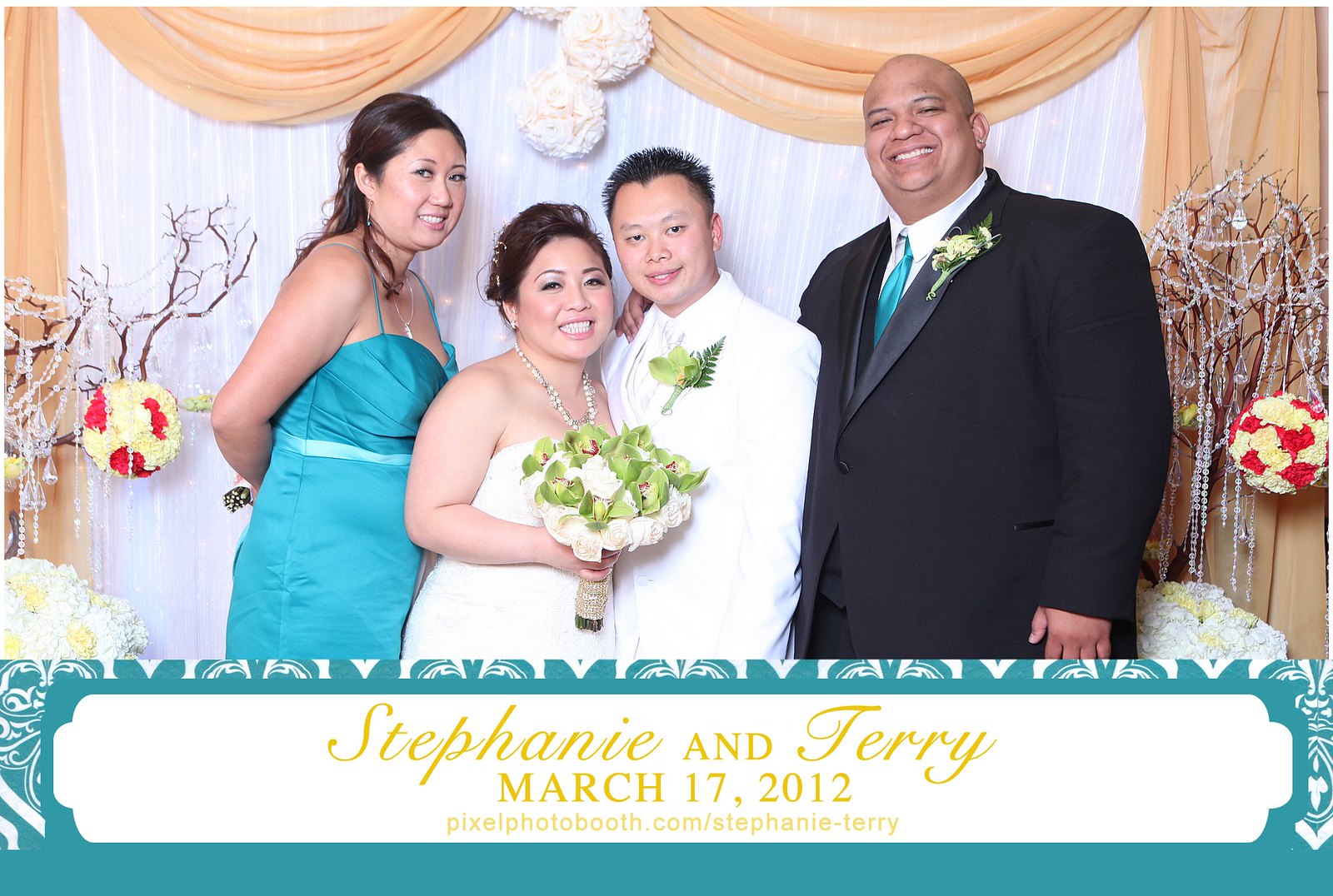The photograph captures a joyous moment from Stephanie and Terry's wedding on March 17, 2012, a day marked by St. Patrick's Day celebrations. The image features four well-dressed individuals standing in front of elegantly draped white and tan curtains, adorned with red and yellow flower balls. From left to right, the first person is a tall woman in a blue silk dress with thin straps, facing sideways but turning her face forward, her long hair cascading down her back. Next to her stands Stephanie, the bride, radiant in a strapless, sleeveless wedding gown and a silver necklace, her hair styled in an elegant updo. She holds a bouquet of green and white flowers, her face forward and beaming with happiness. Beside her is Terry, the groom, distinguished in a white tuxedo with a green floral arrangement on his lapel. He stands facing sideways but looks directly at the camera with a youthful smile. On the far right is a tall, broad-shouldered man of color, wearing a black tuxedo jacket, a white dress shirt, and a blue tie, his face forward and exuding warmth. Their backdrop is enhanced by the sophisticated window drapery and a green banner at the bottom proudly displaying the names "Stephanie and Terry” and the date “March 17, 2012".